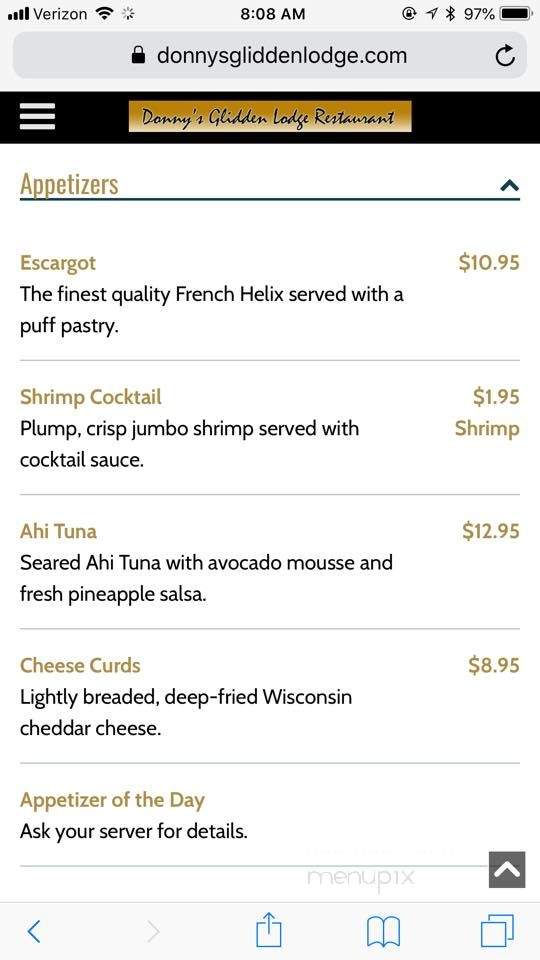**Caption:**

A screenshot of a mobile phone display shows various status indicators at the top, including full Verizon signal strength, Wi-Fi connectivity, loading circle, a time of 8:08 AM, spinning lock indicating orientation is locked, and active location services and Bluetooth. The battery is at 97%. There is a lock icon and the website "Donny's Glidden Lodge.com" is visible. 

A refresh button and hamburger menu are present at the top. The focus of the screenshot is an online menu from Donny's Glidden Lodge restaurant displayed on a dark background with yellow rectangular highlights. The appetizers listed include:

- **Escargot ($10.95):** The finest quality French Helix served with a puff pastry and lime.
- **Shrimp Cocktail ($1.95):** Jumbo shrimp served with cocktail sauce and lime.
- **Seared Ahi Tuna ($12.95):** Ahi tuna with avocado mousse and fresh pineapple salsa, garnished with lime.
- **Cheese Curry ($8.95):** Lightly breaded and deep-fried Wisconsin cheddar cheese, garnished with lime.
- **Appetizer of the Day:** Guests are encouraged to ask their server for more details.

Additional interface elements include an open book icon and a left arrow, suggesting navigation or browsing options within the menu.